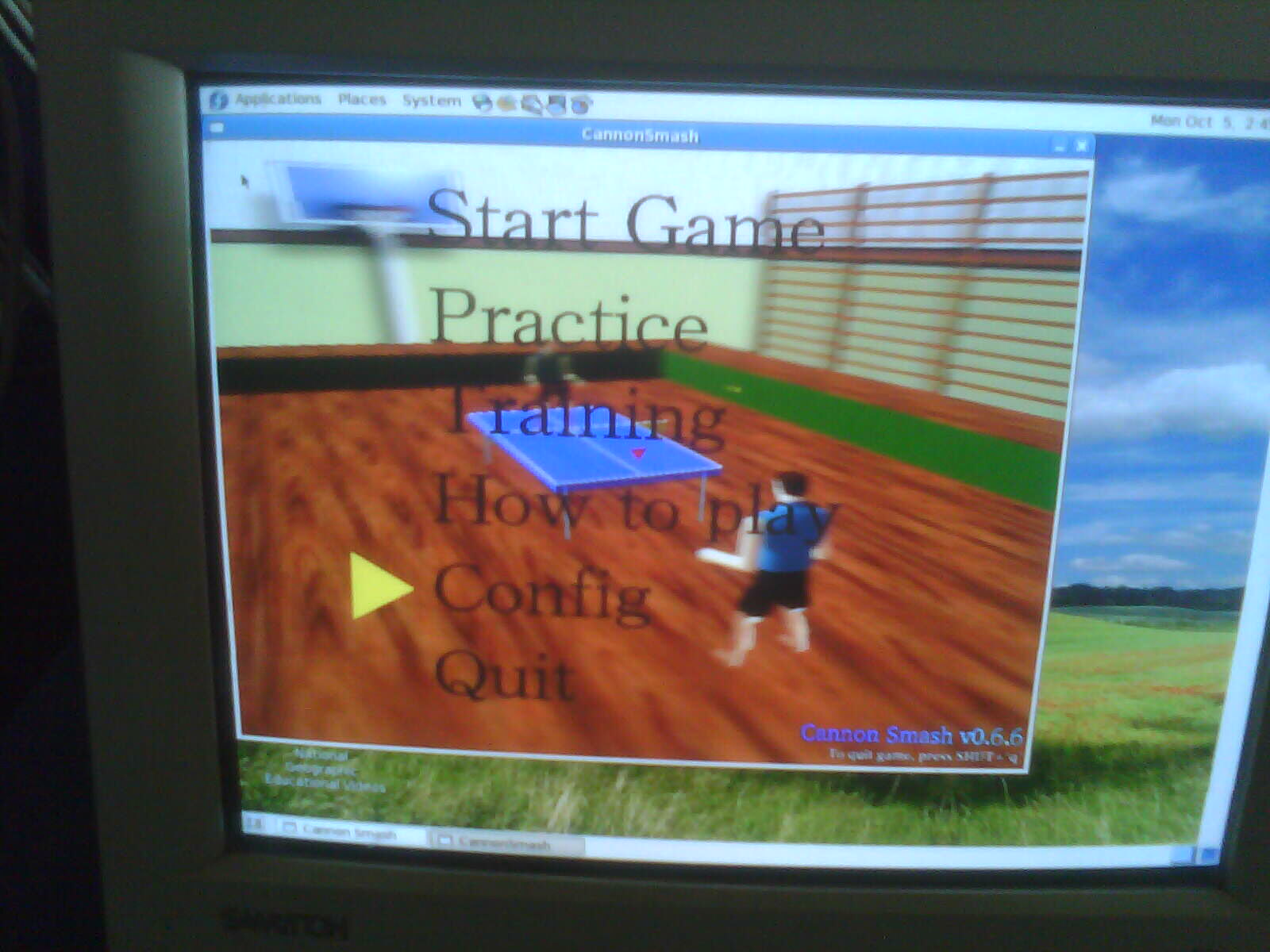The image showcases a slightly curved TV screen, which appears to be a computer monitor projecting a video game interface. The background wallpaper depicts a vibrant scene of blue skies with scattered white clouds above a green grassy field. Dominating the screen is an animated menu for a virtual table tennis game, displayed over a wood-floored room with light green walls and dark green trim. Centrally placed, a blue ping pong table is the focal point of the game interface. The menu options, listed in black text, include: "Start Game" at the top, followed by "Practice," "Training," "How to Play," and "Config," with a yellow arrow pointing to "Config," indicating it’s the current selection. At the bottom, the option "Quit" is displayed. In the bottom right corner of the screen, it reads "Canon Smash version 0.6.6" in blue text.